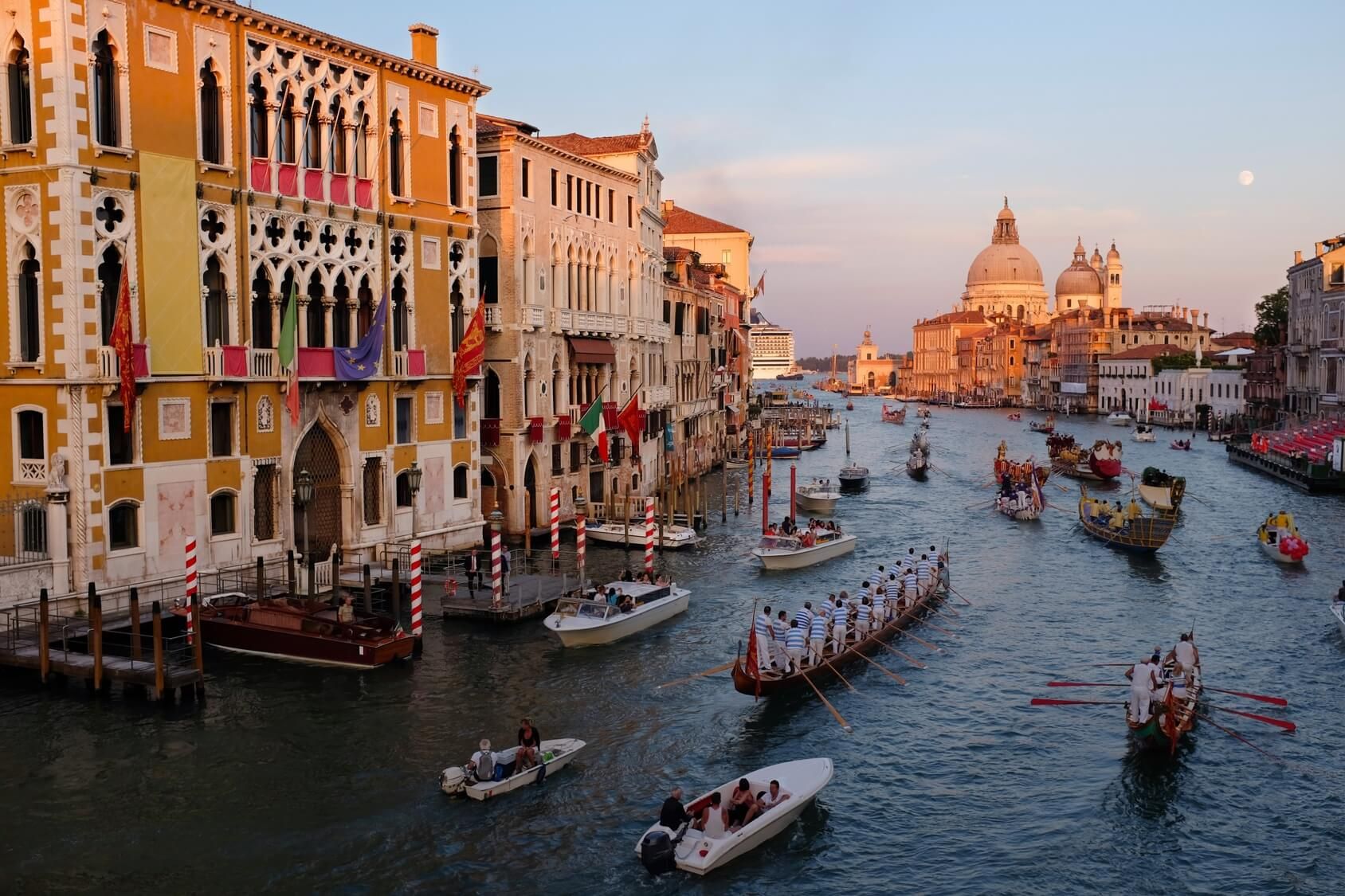The image captures a vibrant canal scene in Venice, Italy, viewed from a balcony in landscape orientation. The bustling canal is filled with an array of boats, showcasing a mixture of traditional Venetian gondolas, paddle-powered vessels, and speedboats. Central to the scene is a large gondola with 16 people standing in white outfits, each holding a paddle. Another prominent vessel, adorned with dragon heads, lies in the bottom right corner, featuring four oars in the water.

On either side of the canal, tall, multi-story buildings with ornate details and colorful exteriors stand proudly. To the left, a bright orange building adorned with colorful flags and black decks for boat docking catches the eye. These buildings display quintessential Venetian architecture, complete with large relief windows and walkways. Docks extend from each building, allowing boats to tie up directly at their bases.

At the far end of the canal, a grand, domed structure rises, adding a touch of regal elegance to the backdrop. The shoreline buildings on the right are equally grand, boasting similar dock setups and intricate architectural designs. Some buildings have outdoor stairs and seating areas, providing spots for people to sit and watch the river activity.

The sky above is light blue, creating a serene contrast to the dynamic, colorful scene below, embodying the essence of Venice’s lively waterways.